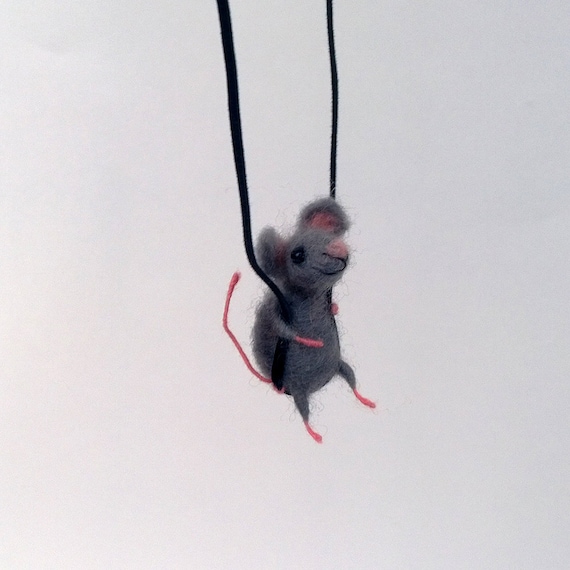The illustration features a charming gray needle-felted mouse sitting on a black shoelace swing against a plain white background. The mouse, crafted with felt material, has a soft and fuzzy texture with small strands of fiber sticking out. It has a pink tail, pink feet, pink inside its ears, and a pink nose. The mouse's big black eyes, possibly sewn or knitted onto its felt body, add to its endearing expression as it smiles, showcasing a bit of black thread representing its mouth. It grasps the swing's ropes with its front legs, which are positioned like arms, while its back legs dangle off the swing's edge. The black shoelace swing is suspended from an unseen support above the frame. Overall, it's an adorable and intricately detailed craft project capturing a playful and whimsical scene.